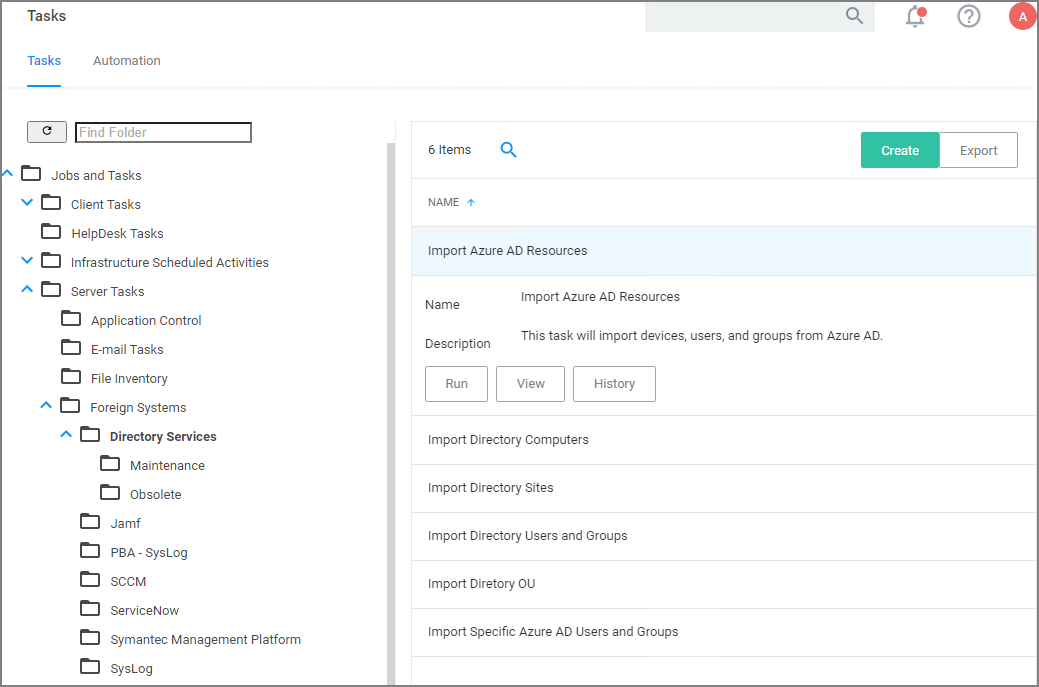The image in question is a detailed screenshot of what appears to be a software application or directory interface, possibly for task management or system automation, displayed on a computer screen. The layout features a simplistic design with black and gray text on a white background, creating a clean and easily readable display.

On the top left corner of the interface, the word "task" is visible. The top right corner contains several icons: a search box, an alerts icon with a red dot suggesting there are pending alerts, a help icon represented by a circle with a question mark, and a red circular icon with a white "A" inside, the function of which is unclear.

Below the top bar, there are two menu tabs. The "Tasks" tab is blue, indicating it is currently active, while the "Automation" tab is grayed out. Beneath these tabs on the left side, a search field labeled "Find Folder" with an adjacent activation button is present.

The left column of the display shows a hierarchical structure of folders and subfolders, starting with a main folder labeled "Jobs and Tasks." Nested under this main folder are several subfolders: "Client Tasks," "Help Desk Tasks," "Infrastructure Schedule Activities," and "Server Tasks." The "Server Tasks" folder itself contains additional nested folders, demonstrating a multi-tiered system of organization. In total, the complex structure seems to comprise approximately 2,000 folders and subfolders.

The right side of the interface features various interactive elements: a search box, a field for a user's name, and a link labeled "Import Azure AD Resources" highlighted in blue text. Below this link, several buttons are available, including "Run" and "View History," accompanied by other unspecified lines and interactive options, which complete the interface's layout.

Overall, the interface serves as a comprehensive and organized directory for managing multiple categories of tasks and automation processes.